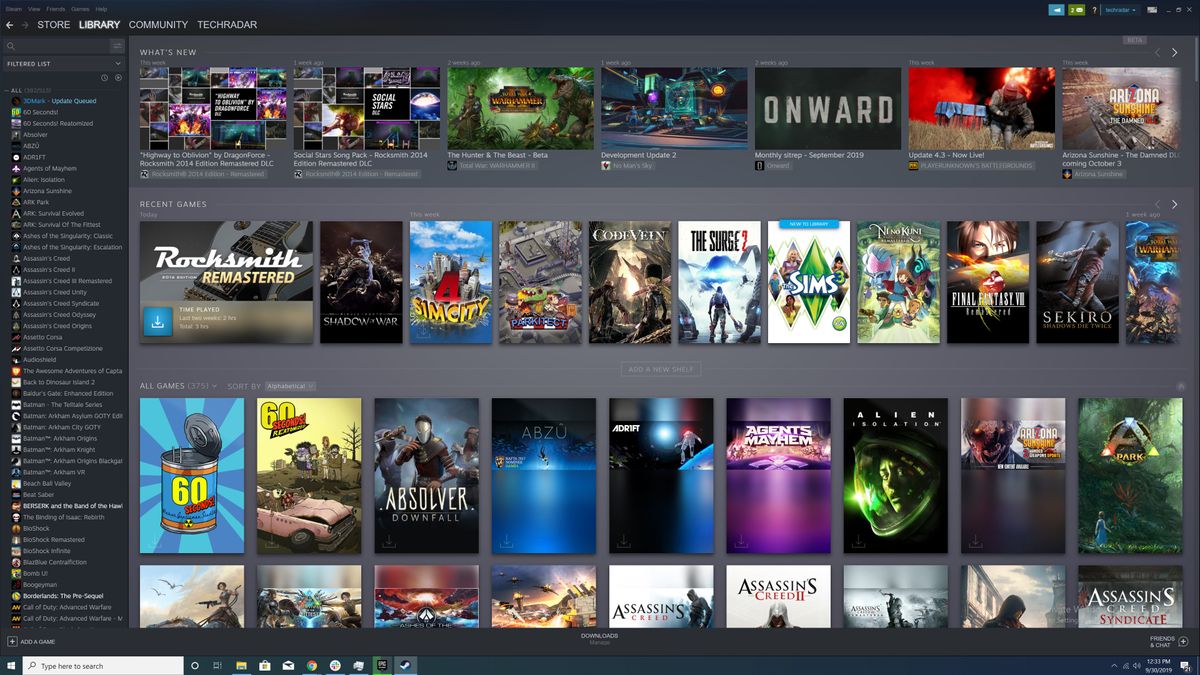This screenshot appears to be from the Steam client interface. It showcases the Library section, as indicated by the bold and white-highlighted "Library" tag at the top left, among other tabs such as Store, Community, and TechRadar.

On the left pane, there is an extensive list of contacts or messages. The first item on this list is distinguished by blue text and reads "3QMarkUpdateQueued." The list extends with over 20 such entries visible.

To the right, the main content of the screenshot is divided into several sections. The "What's New" section highlights recently updated or added content on Steam, featuring seven entries: 
1. "Highway to Oblivion"
2. "Social Stars Song Pack"
3. "The Hunt and the Beast"
4. "Development Update 2"
5. "Monthly Street"
6. "Now Live"
7. "Arizona Sunshine"

Below that, the "Recent Games" section lists games that have been recently accessed. Recognizable titles include:
1. "SimCity 4"
2. "Shadow of War"
3. "The Surge 2"
4. "The Sims 3"
5. "Final Fantasy 7"

Lastly, the "All Games" section offers a broader view of available games in the user's library which consists of:
1. "Absolver"
2. "Agent Mayhem"
3. "Assassin's Creed 2"
4. "A Park"

The layout provides a comprehensive glimpse into the user's Steam library and recent activity.